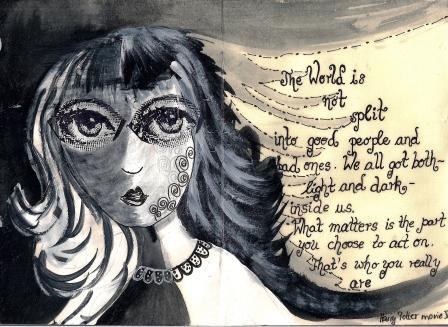The image is a detailed black and white drawing of a woman with striking, dual-colored long wavy hair—black on the right side and white on the left side. Her hair, adorned with intricate curls, cascades down to her shoulders, although the image itself is cropped at her shoulders, concealing any clothing detail. Her face, depicted with precision, displays small thin lips, large expressive eyes with makeup, and jewelry intricately drawn onto her skin. She also sports short bangs that delicately frame her forehead and a delicate necklace around her neck. The woman's face is divided with a shadow effect, creating a stark contrast: the left half appearing darker while the right half is lighter. This artistic piece of work, reminiscent of a watercolor graphic, features a muted background—black on the left and tan on the right, which enhances the visual split. To the right of the woman, within the tan background, a thought-provoking quote in cursive reads, "The world is not split into good people and bad ones. We all got both light and dark inside us. What matters is the part you choose to act on. That’s who you really are."